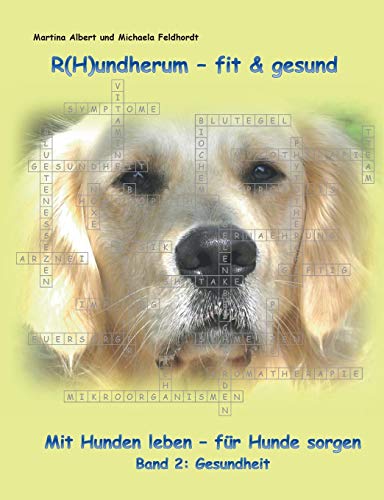The poster features a solemn Golden Retriever with long, shiny golden fur on its ears and a grayish-white face. The dog's mouth is closed, and it has a sad expression. The backdrop of the image is a light yellow hue, and the center of the layout features a translucent crossword puzzle overlaying the dog's face, filled with various words associated with dog care. At the top of the poster, the title reads "R-H-U-N-D-H-E-R-U-M - fit and decent" in bold blue font. Just below this title, in smaller black letters, it states "Martina Albert und Michaela Feldort." The bottom section of the poster contains foreign text in blue, reading "M-I-T-H-H-U-D-N-L-E-V-E-N - für Hundesorgen," followed by "Bantu: [colon]."